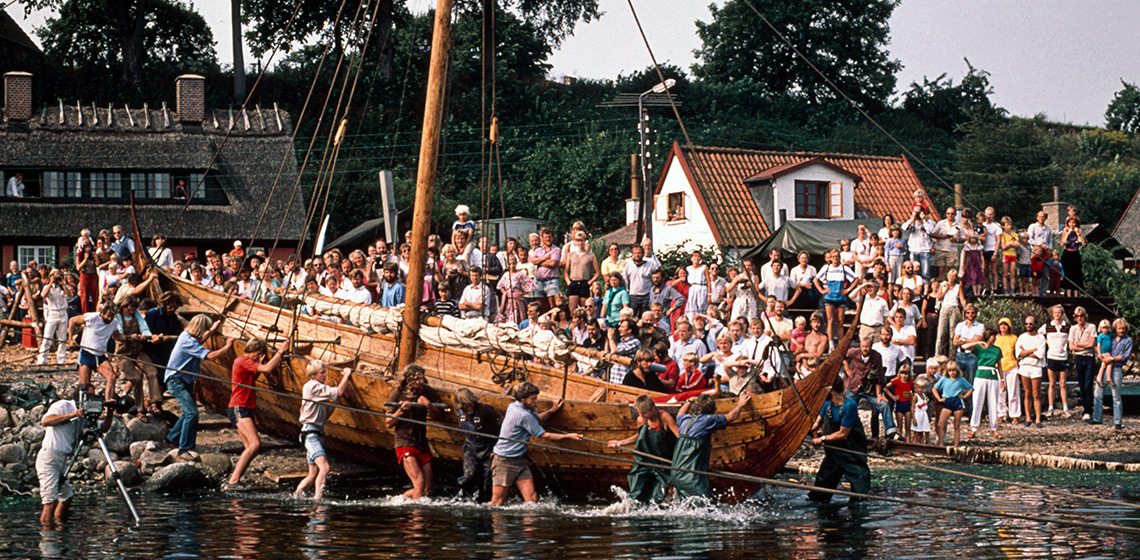In this vibrant outdoor scene, a bustling crowd of about 100 to 200 individuals is gathered around a wooden, old-style ship at a marina, likely in Europe due to the presence of traditional clay-roofed houses seen in the background. The clear sky and lush green trees suggest it's spring or summer. The ship, resembling a large canoe or possibly a sailboat, is actively being pushed into the water by 10 to 20 dedicated individuals who are gripping its edges and pulling on a line or cord. Many people are also in the boat, splashing in the shallow water around it. Additionally, numerous onlookers are capturing the moment with their cameras, hinting at a possible movie scene, evidenced by a person with a camera on a tripod in the lower left corner of the image. Behind the crowd, rows of houses with varying roof styles are partially obscured by both the people and the abundant trees. A tall pole with several lines extends from the boat, suggesting it may have been a sailboat, although no sail is visible. The image captures a lively, communal effort and a historic ambiance.